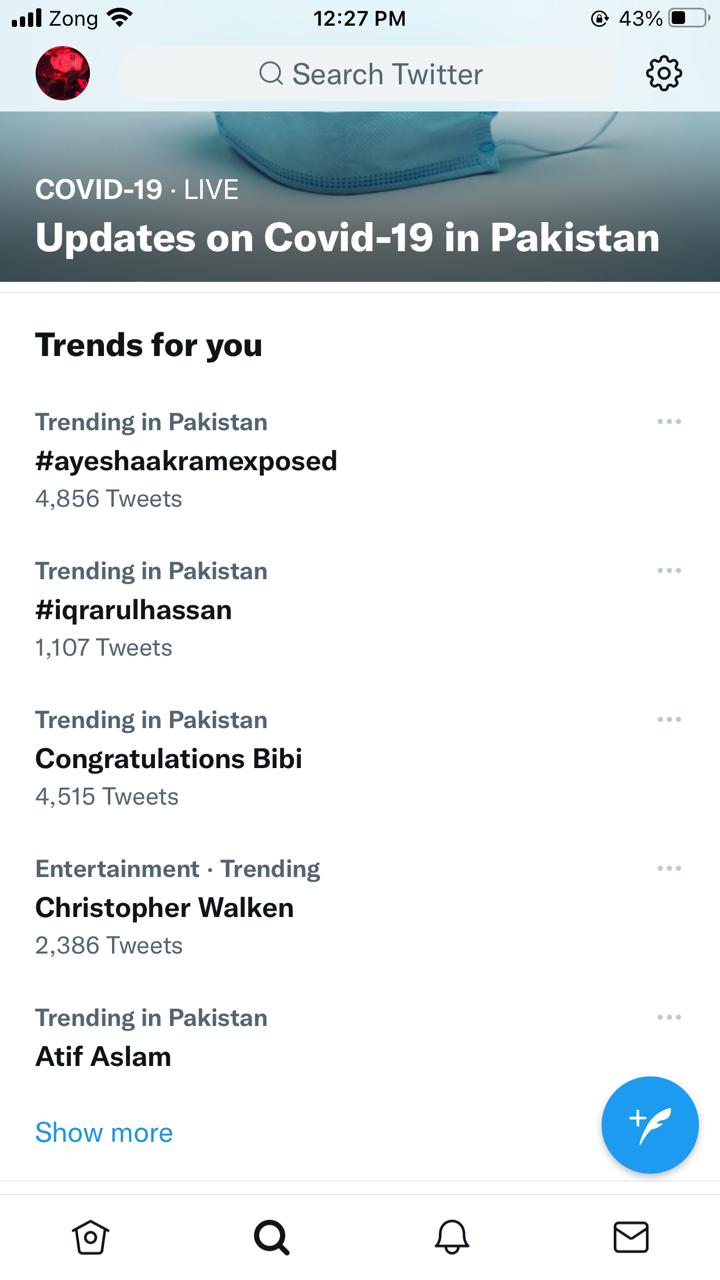A detailed screenshot of a Twitter interface captured at 12:27 PM with a 43% battery level, displayed on a white background. At the top, there is a light blue "Search Twitter" field. To the left, there's an icon with a red and black circle—potentially a user's profile picture, though it's indistinct. A gear menu icon is positioned to the right of the profile picture. Below, a prominent update features a JPEG image displaying "COVID-19 live" and "Updates on COVID-19 in Pakistan," with a blue face mask laid on a white surface.

Following the update, the "Trends for you" section highlights various trending topics in Pakistan:
1. "**Ayesha Cram Exposed**" – 4,856 tweets.
2. "**Iqraul Hassan**" – 1,107 tweets.
3. "**Congratulations Bibi**" – 4,515 tweets.
4. "**Christopher Walken**" (Entertainment trending) – 2,386 tweets.
5. "**Atif Aslam**"

Each trending item is in bold black text, contrasting with the lighter gray of supportive text. At the bottom of the trends list is a blue "Show more" link. Adjacent to this, there's a blue circle with a feather icon and a "+" sign.

Towards the lower section of the screenshot are four icon-only buttons for Home, Search, Notifications (bell), and Direct Messages (email).